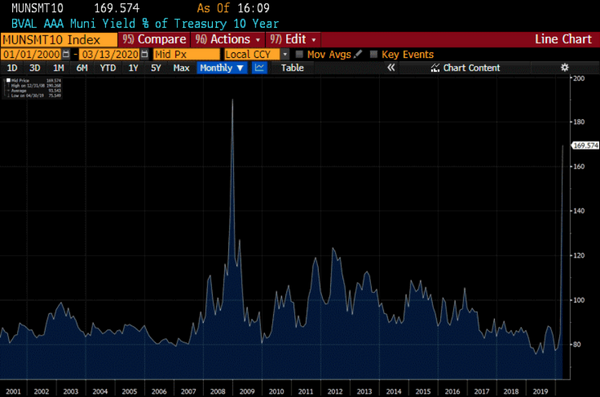This image captures a detailed screenshot of financial data, likely related to stock markets or bond yields. At the very top of the screen, the text reads "MUNSMT." The predominant feature is a line graph that spans from 2001 to 2019 along the horizontal axis. The vertical axis, positioned on the right side, ranges from 80 to 200, marked at intervals of 20.

The line graph's background is shaded blue, with the data points highlighted in white for better visibility against the dark background. Above the graph, teal text displays various financial terms, including 'BV,' 'ALA,' 'Muni Yield,' and 'Treasury 10 Year.' Additional labels, such as 'Munis 10 Index,' are present, each accompanied by red rectangular markers, adding emphasis to specific parts of the data. The screen is filled with numerous numbers and letters, providing a complex yet comprehensive overview of the financial trends being analyzed.